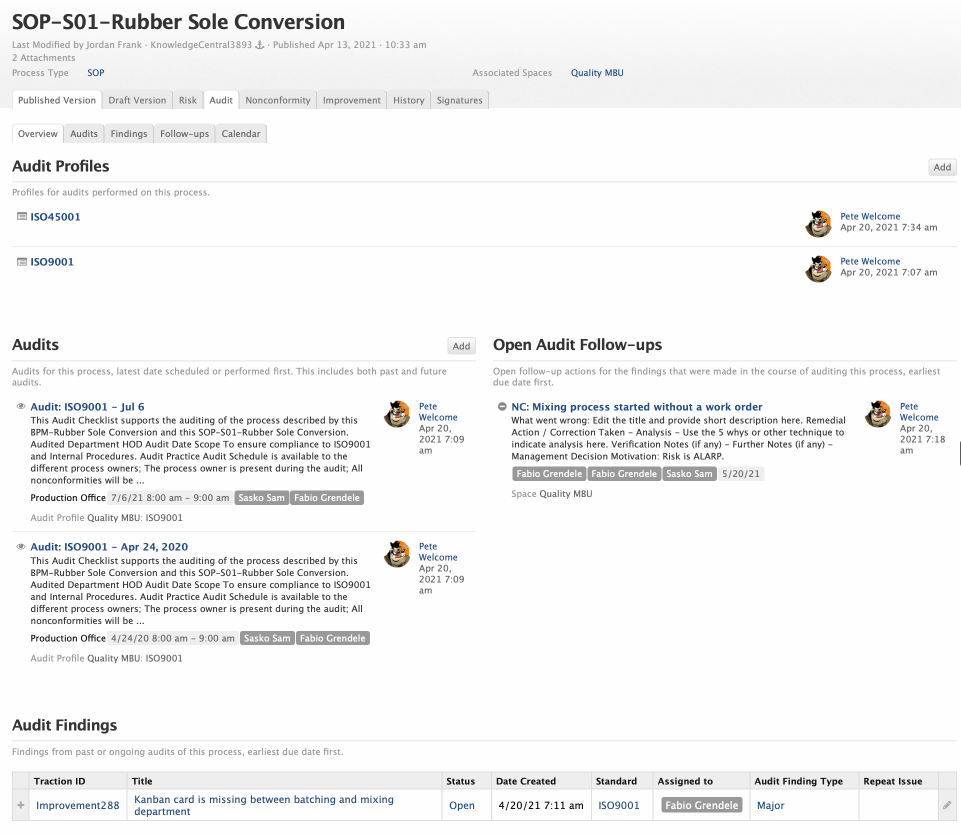**Detailed Caption:**

The image features a light blue background with detailed content related to SOP-SO1 rubber sole conversion. At the top, a header reads "SOP-SO1 Rubber Sole Conversion," followed by small text in process type that includes terms like SOP and associated spaces, quality, and MBU. 

Just beneath the header are multiple tabs labeled: "Published Version," "Draft Version," "Risk," "Audit," "Nonconformity," "Improvement," "History," and "Signatures."

Below these tabs, there is a section titled "Audit Profiles," featuring a white box with some identifiers and an image. The first box includes the ID "1504-5001," an image, and text reading "Pete Welcome, April 20th, 2021, 7:34 a.m." Alongside it, there is an "Add" button. Another box follows with the ID "1509-001," also containing an image and reading "Pete Welcome, April 20th, 2021, 7:07 a.m."

Under the "Audits" section, there is an icon resembling a small 'i' for "audit," along with a date "July 6th," and beneath it are two small buttons. Another audit entry displays with the date "April 24th, 2020," labeled "Production Office," and flanked by buttons and images of Pete Welcome.

On the right side of the image, the "Open Audit Follow-Ups" section includes a gray circle with a white line. It states, "NC mixing process started without a work order," with another image of Pete Welcome and three gray buttons beside it.

At the bottom lies the "Audit Findings" table with headers "Traction ID," "Title," "Status," "Date Created," "Standard," "Assigned To," "Audit Finding Type," "Repeat Issue." One of the entries lists "Improvement 288" indicating that a "Kanban card is missing between batching and mixing department," with status "Open" as of "2021, 7-11 a.m.," under "ISO 9001," assigned to Fabio Grindale, classified as a "Major" issue.

This detailed layout captures the various elements and data points presented in the image, providing a comprehensive overview of the rubber sole conversion process and associated audit details.